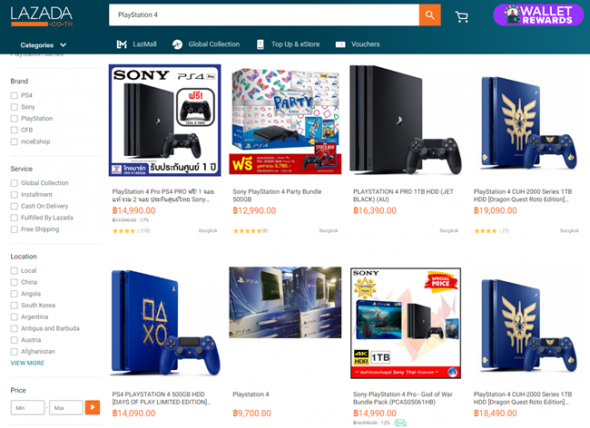The image features a bustling e-commerce webpage from Lazada. In the upper left corner, the Lazada logo is clearly visible, followed by an orange bar labeled "CO.TM." Just below it, the search field shows the term "PlayStation 4" and is accompanied by an orange search button on the right. Adjacent to this is a purple button labeled "Wallet Rewards" alongside a shopping cart icon.

Running along the top is a dark teal band that contains several dropdown menus. These include options labeled "Categories," "LazMall," "Global Collection," "Top-Up & eStore," and "Vouchers" all written in white. The white background below this band showcases a grid of items arranged in a 4x2 format.

In the upper left of this grid, a listing for a "Sony PS4 PlayStation 4 Pro" is displayed, priced at $14,990. The item appears to have a rating, but the resolution makes it unclear. Beside it, another listing shows a "Sony PlayStation 4 Party Bundle" priced at $12,990 with what appears to be a five-star rating. The overall resolution of the image is moderately poor, making some details hard to discern.